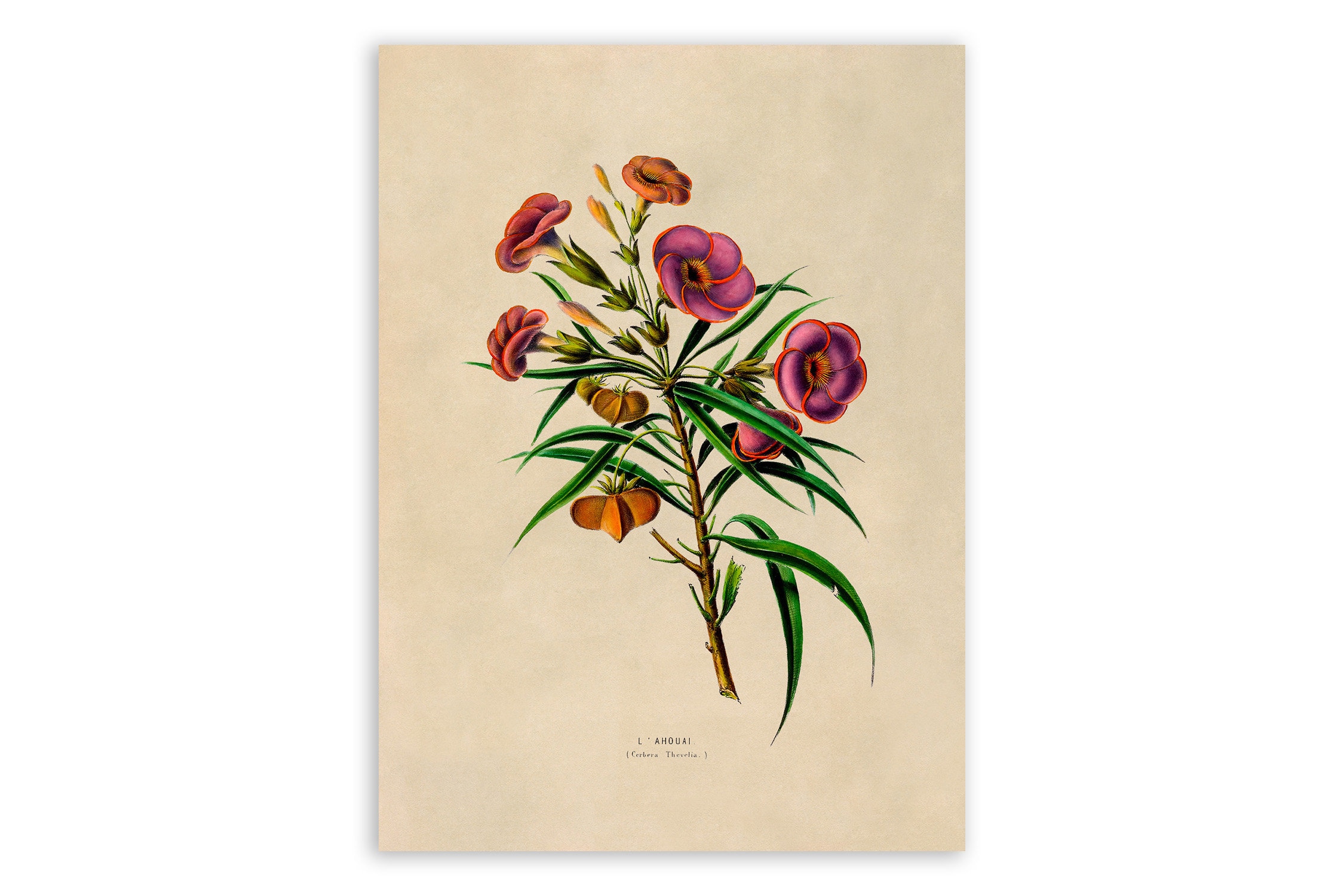A detailed Victorian-style color sketch on yellowed, off-white paper portrays a vertically oriented sprig of a flowering plant. The artwork meticulously depicts a green stem with long, pointed, dark green leaves. Various flowers emerge from the stem, including vibrant pinkish-red blossoms and orange-hued flowers. Notably, there are also a few unopened yellowish bulbs near the top. The plant is likely drawn from a bush, given the abundance of leaves and flowers. At the bottom of the page, partially legible black text appears, reading "L----- a M o u r i", with smaller text below, possibly indicating the Latin name of the species. The page suggests it comes from an old, weathered book.